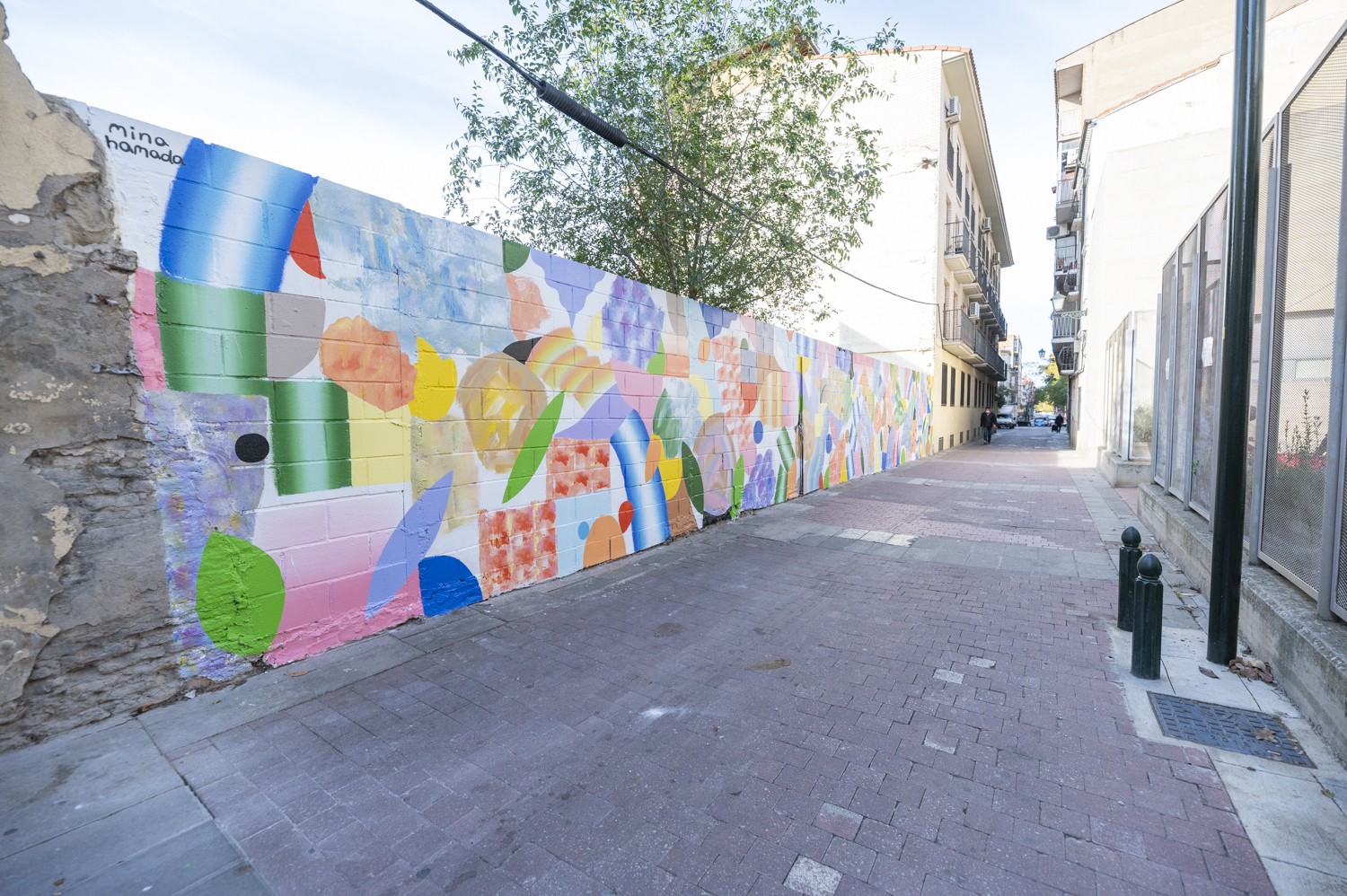The image depicts a vibrant and colorful mural sprawling across a large cinder block wall, reminiscent of those found in narrow city alleyways. The mural, which likely transformed an otherwise plain brick wall, is rich with bright, electrifying colors such as electric blue, bright green, lime green, bright orange, and bright red. It features a diverse array of shapes including cubes, ovals, surfboard-like forms, as well as more abstract patterns resembling leaves, quilt squares in pink and peach, and sections that mimic sky with blue and white clouds. 

The mural, credited to an artist named Mina Hamada, spans the length of the alley, bordered by a brick walkway and accompanied by glass windows that suggest a nearby shop or potential greenhouse. A black lamp post and overhead electrical cord are also visible in the scene, adding to the urban atmosphere. In the background, a lush tree peeks out, enhancing the mural's joyful and eclectic aesthetic.